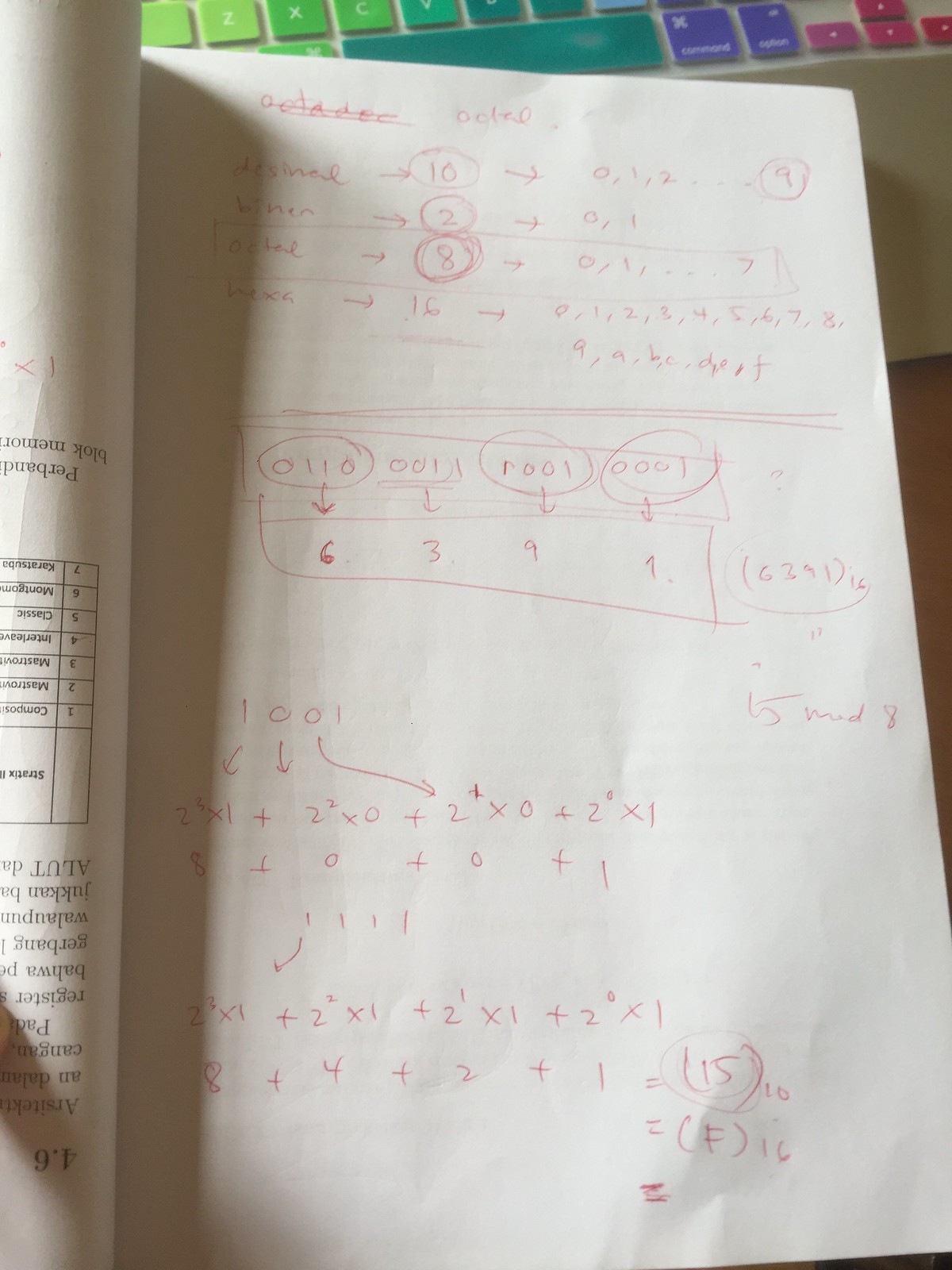This photograph captures a workspace, providing a top-down view of a workbook and a computer keyboard. The keyboard at the top of the image showcases a gradient of colors, beginning with light celery green keys on the left, transitioning into deeper greens, blues, and culminating in a teal space bar. The array also includes deep purple, violet, and red keys set against an ivory background.

In the foreground is an opened workbook. The left page, folded back and positioned upside down, features the heading "4.6" at the top, with partial sentences and a table just below. Meanwhile, the right page is entirely visible, filled with handwritten equations and calculations. Some numbers and equations are circled for emphasis, all penned in a faint purple ink. This detailed view highlights both the colorful and organized aspects of the user's study environment.